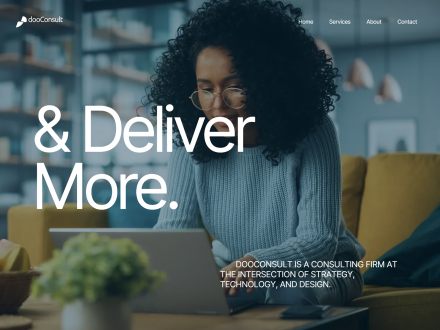This image is a cropped screenshot of the DoConsult home page as viewed on a desktop browser. The background features a photograph of a woman sitting comfortably on a couch, engaged with a laptop. In the top-left corner, the DoConsult logo is prominently displayed in white. Opposite the logo, in the top right, the website’s navigation menu is visible in small white text, listing categories such as Home, Services, About, and Contact. Centralized on the left, a bold and large white text reads "Deliver More," capturing immediate attention. Towards the bottom-right, in small uppercase white letters, an informative tagline states, "DoConsult is a consulting firm at the intersection of strategy, technology, and design." The remainder of the page is cropped out, focusing the viewer’s attention on the key elements described.